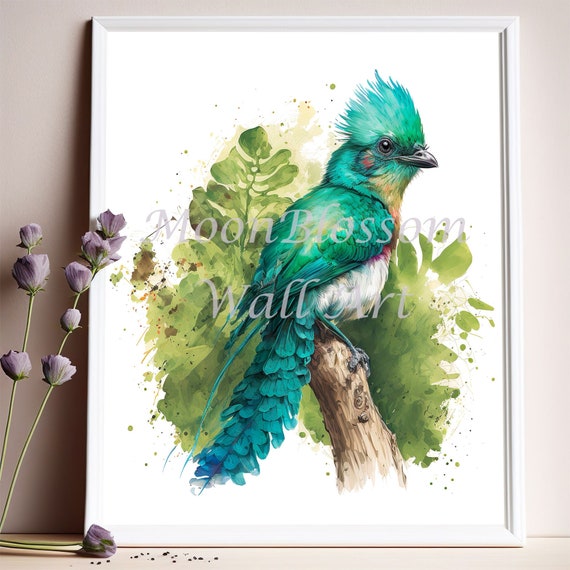The painting, propped up on a beige mantle, is framed in a whitish-gray frame and features a striking turquoise bird with black eyes and a black beak, perched gracefully on a branch. The bird, centered in the composition, has long, layered tail feathers and distinctive tufts on its head resembling a teal mohawk. Its vibrant plumage includes accents of blue, yellow, red, and white, with a notable splash of yellow on its neck. Behind the bird, green leaves are meticulously illustrated against a clean white background. Complementing the scene, delicate purple flowers with green stems are arranged decoratively to the left, enhancing the lively, realistic feel of the painting.